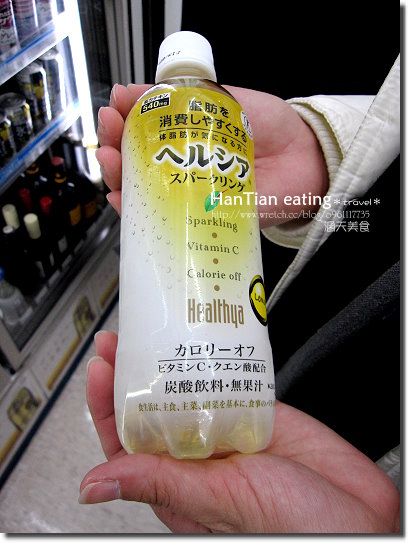In the photograph, a person is holding a bottle of a health drink with both hands, with one hand on the bottom and the other on the top. The person is dressed in a white jacket over a white shirt and appears to be wearing a black scarf on their right side. The bottle, which has a white twist-off plastic cap, features a plastic label with both Japanese and English text. The label transitions from white to yellow, delineating the gradients from lighter to darker shades of yellow. The English text prominently displays words like "sparkling," "vitamin C," "calorie off," and "health yeah." There are also segments of Japanese text, particularly towards the bottom, indicating that it is a lemon-flavored drink. In the top left corner of the background, there's a refrigerator or cooler stocked with various bottled drinks and cans, alongside shelves with plastic pieces marked by blue lines. The image foreground also includes text like "hantin," "eating," and "travel" with ampersands, suggesting a possible website address starting with "HTTP." The floor in the bottom left corner is composed of white and grayish tiles.